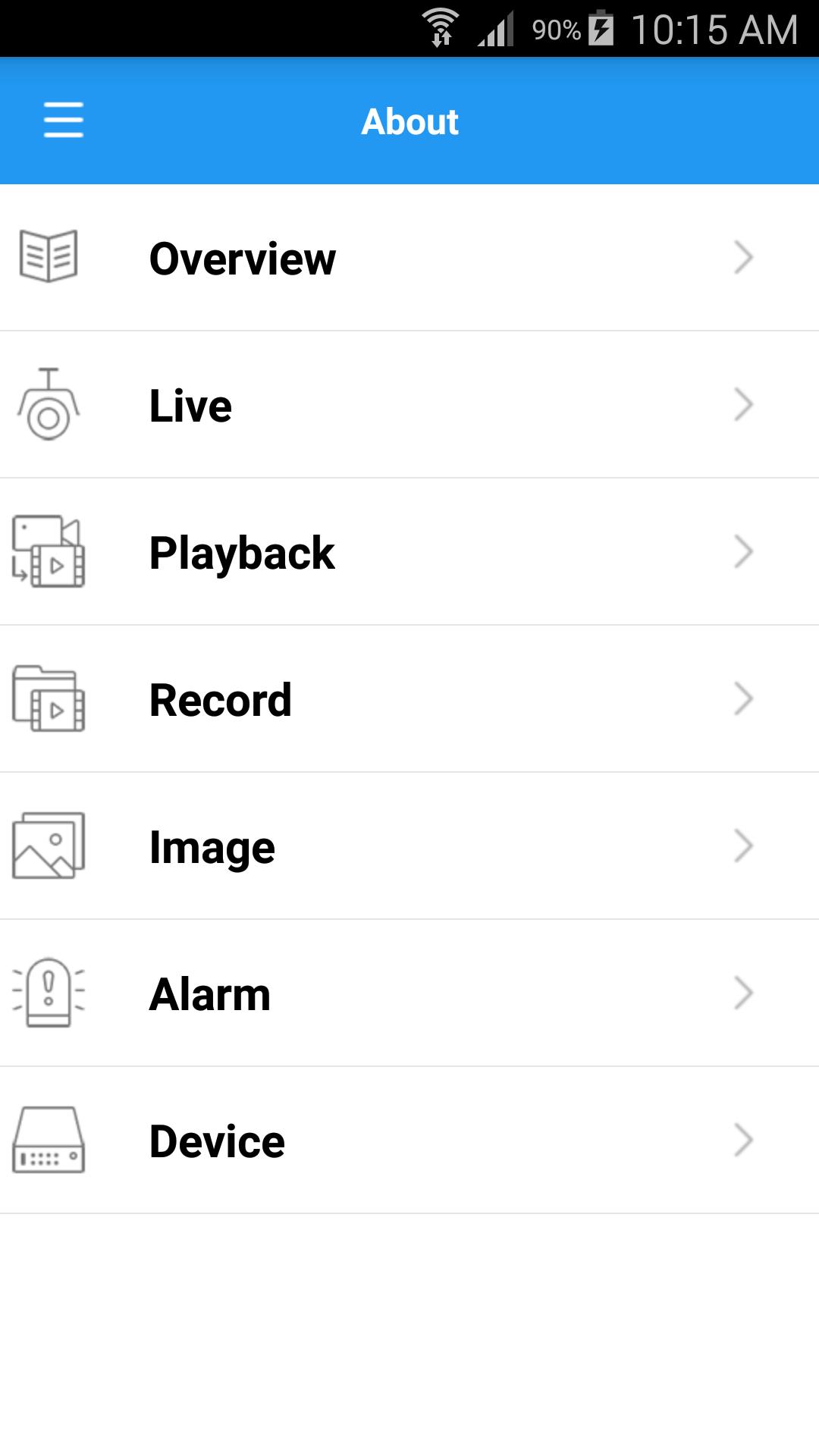This is an image of a smartphone screen displaying the 'About' page within an application. At the top of the screen, a thin black bar shows the time (10:15 a.m.), the battery status (charging at 90%), and other typical status icons. Below this is a thicker blue rectangle with the word 'About' prominently displayed in white text. To the left of the word 'About' are three horizontal white lines, indicative of a menu icon.

Beneath the blue rectangle, there are various options listed: 'Overview,' 'Live Playback,' 'Record,' 'Image,' 'Alarm,' and 'Device.' Each option is written in black text and accompanied by a white icon that visually represents its function. These labels are separated by faint gray lines. To the right of each option is a column of arrows pointing to the right, suggesting that these options are navigable or expandable for more information.